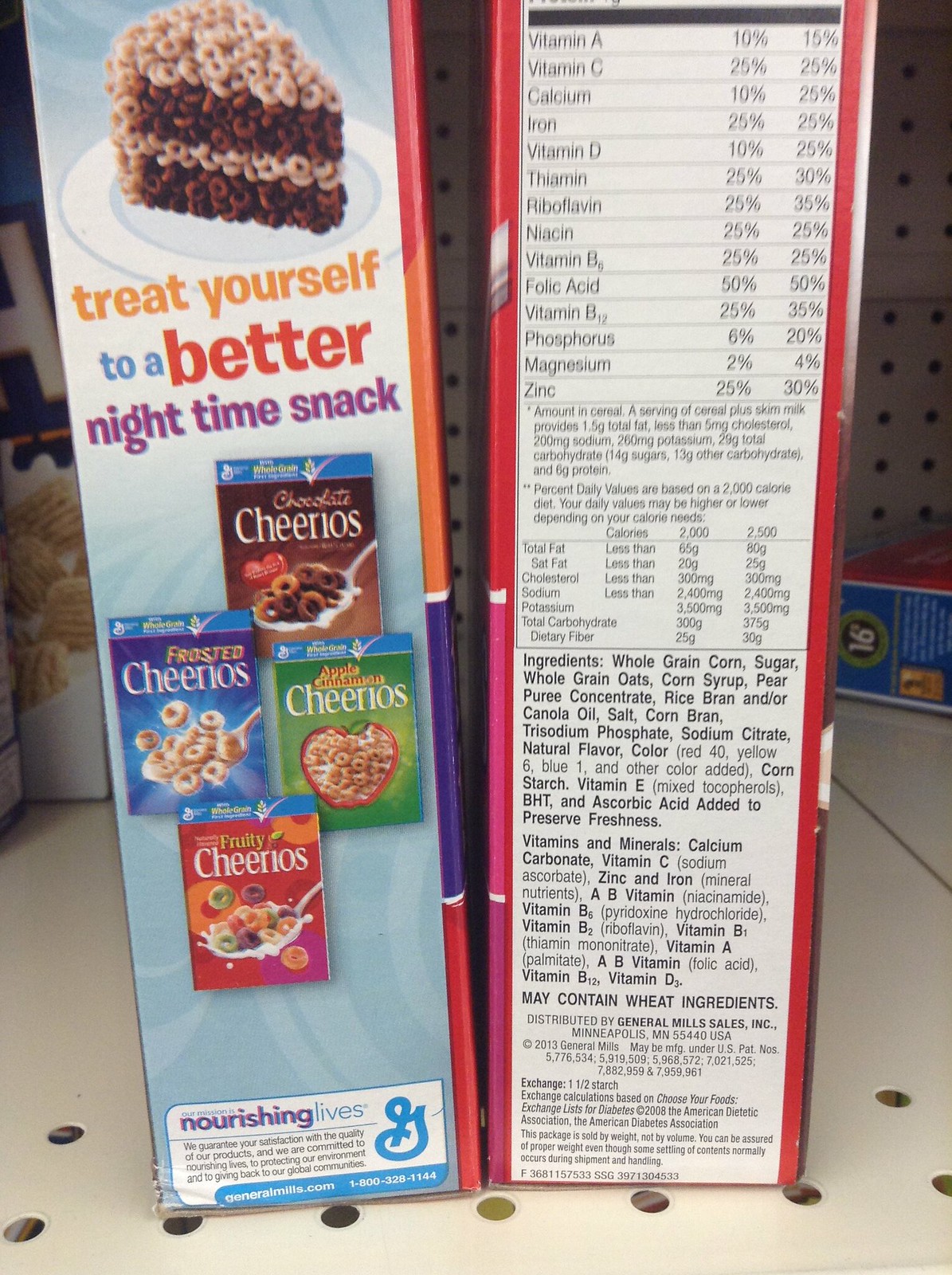In this vertically-oriented photograph, we see two cereal boxes standing upright on a supermarket shelf, viewed from the side. The box on the left showcases four varieties of Cheerios: Chocolate Cheerios, Frosted Cheerios, Apple Cinnamon Cheerios, and Fruity Cheerios. Above these four boxed images, there is a depiction of a slice of pie or layer cake assembled from Cheerios, with light-colored Cheerios on top and dark-colored Cheerios in the center. The text above the image reads, “Treat Yourself to a Better Nighttime Snack.” The box on the right displays nutritional information and ingredients. Nutritional details include Vitamin A at 10%, Vitamin C at 25%, Vitamin B12 at 25%, and Folic Acid at 50%. The list of ingredients comprises whole grain corn, sugar, whole grain oats, corn syrup, pear puree concentrate, rice bran, salt, and corn bran.